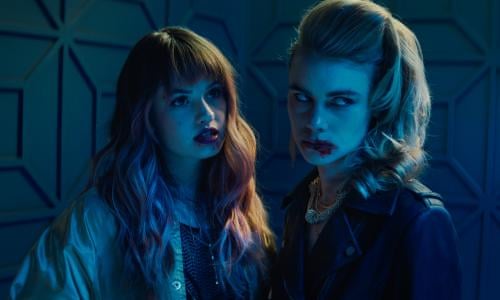In the dimly lit image, bathed in a bluish hue, two young women with pale complexions stand side by side, exuding a sinister aura. The girl on the left has long, wavy auburn hair with straight bangs that lightly graze her forehead. She is dressed in an open button-down shirt over a black top, the edges of her lips smeared with what appears to be either blood or lipstick, contributing to a disheveled and eerie look. Her gaze is directed slightly upwards to the right, as if she’s fixated on something unseen.

To her right stands another girl with a menacing look, her mouth clearly smeared with blood, hinting at a recent, gruesome act. She has her blonde hair styled in a high, poofy ponytail and wears a black leather biker jacket, which enhances her intimidating presence. Her head is tilted slightly as she glares off to the side, her expression cold and unforgiving.

The backdrop of the image features structures akin to those found in a medieval castle, with geometric lines adding to the overall dark and foreboding atmosphere. The interplay of bluish light and shadow makes the scene even more grim, solidifying the impression that these young women may be vampires, lost in their macabre world, and possibly caught in the aftermath of a nightmarish event.